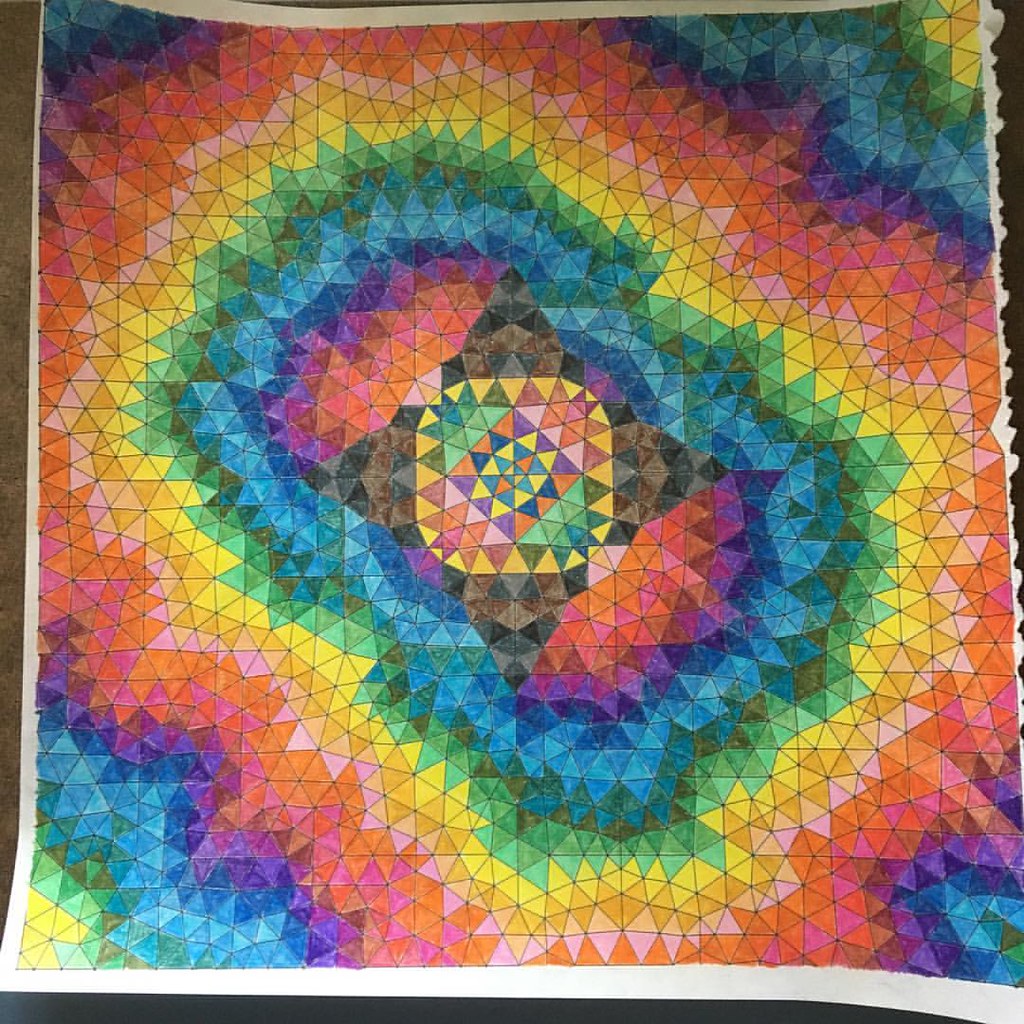The image depicts an intricate piece of art that appears to be crafted on a textured surface, possibly paper or fabric. The artwork is not entirely flat but instead rests on a dark, possibly brown, hard surface. This visually compelling piece is composed of numerous small panels, primarily triangles, which collectively form vibrant color patterns across the image.

The edges of the artwork are distinctly segmented: the top left corner features a deep blue, the top right shines with bright yellow, the bottom right merges shades of blue and green, while the bottom left combines blue, green, and yellow hues. Within these edges, a series of concentric rings showcase a diverse palette of colors, ranging from pinks and purples to oranges, deep and light yellows, light and deep greens, and various shades of blue. Towards the center of the composition, the colors intermingle more freely, creating a dynamic and eye-catching mosaic of myriad hues.